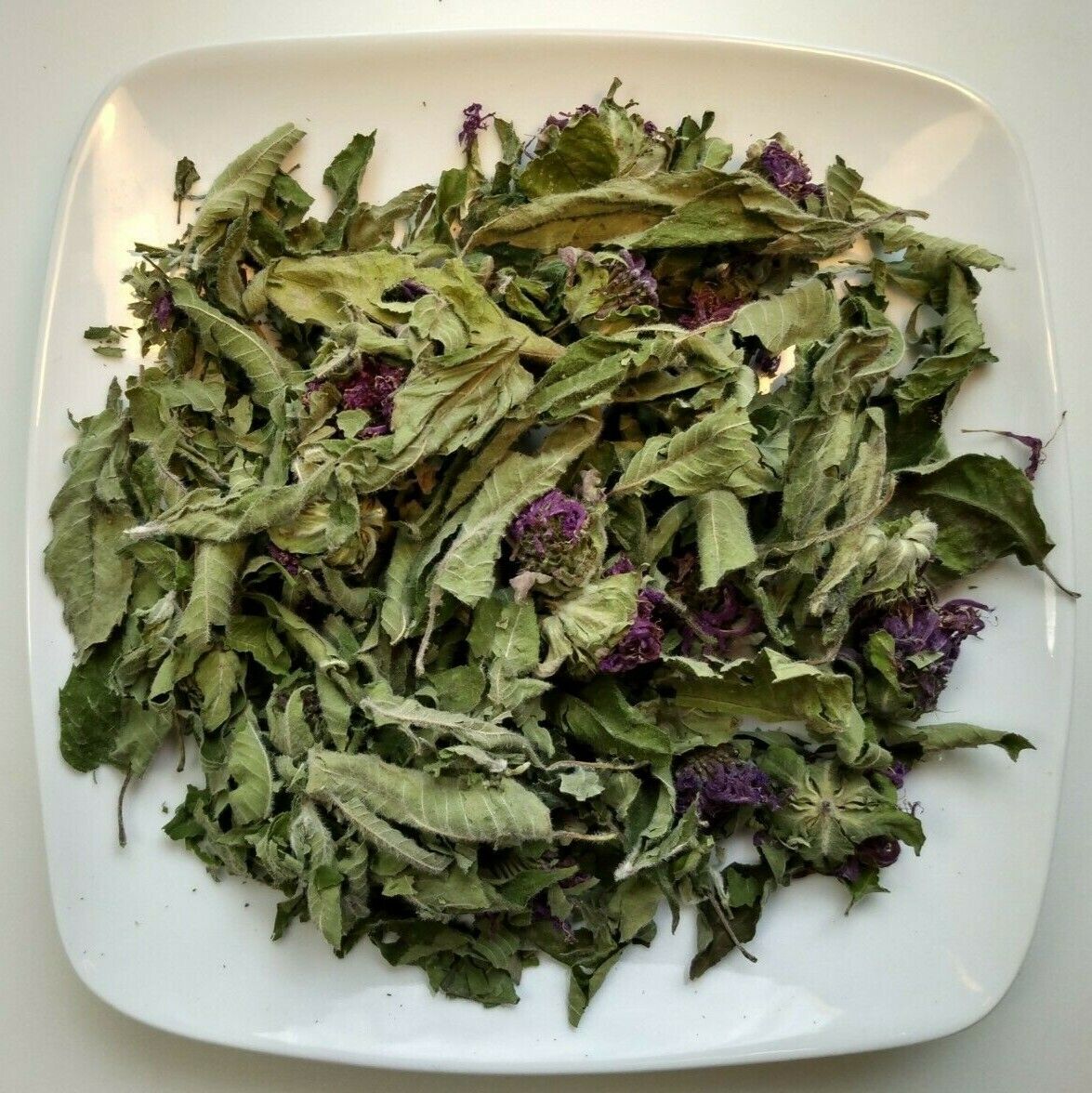The image depicts a large, square ceramic plate with curved corners and a glossy white finish, resting flat on a white surface. The plate is covered with a pile of dried leaves, mostly green and shriveled, curling inwards and exhibiting signs of decomposition. Among the green leaves, there are sprigs of purple leaves and a few dry, hard stems. Some leaves are flipped, revealing their white veins. The overall appearance of the leafy pile is unappetizing and very dry, looking as though they could easily crumble to the touch. Only the small edges of the plate are visible, accentuating the abundance of the dried foliage.